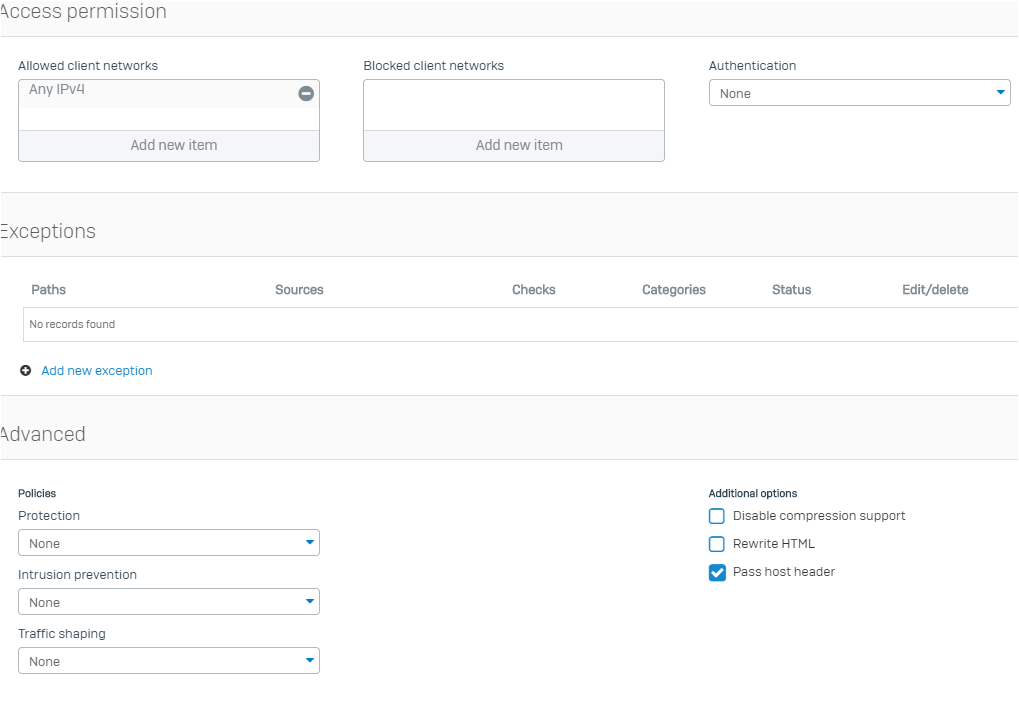The image depicts a detailed interface of a website that appears to function as a file entry or client management system, potentially for an insurance agency or similar professional services. The interface features several sections with specific fields and options:

- **Access Permissions**: 
  - **Allowed Client Networks**: Any IPv4.
  - **Blocked Client Networks**: None listed.
  - **Authentication**: None.

- **Exceptions**: 
  - **Current Records**: No records found.
  - **Related Subtext Options**: Sources, checks, categories, and status – all currently empty.
  - **Add New Exception Button**: Highlighted in blue.

- **Advanced Settings**: 
  - **Policies Section**: 
    - Three dropdown menus:
      - **Protection**: Set to none.
      - **Intrusion Prevention**: Set to none.
      - **Traffic Shaping**: Set to none.

  - **Additional Options**: Located on the bottom-right side:
    - Three checkboxes:
      - **Disable Compression Support**: Not checked.
      - **Rewrite HTML**: Not checked.
      - **Pass Host Header**: Checked, marked with a blue checkmark.

Most of the text is displayed in traditional black over a white and gray background, giving a clean and professional appearance to the interface. The primary interactive element, the "Add New Exception" button, is distinctly marked in blue, drawing attention to it amidst the otherwise monochromatic color scheme. This suggests an IP management or user permissions configuration setup on the website.